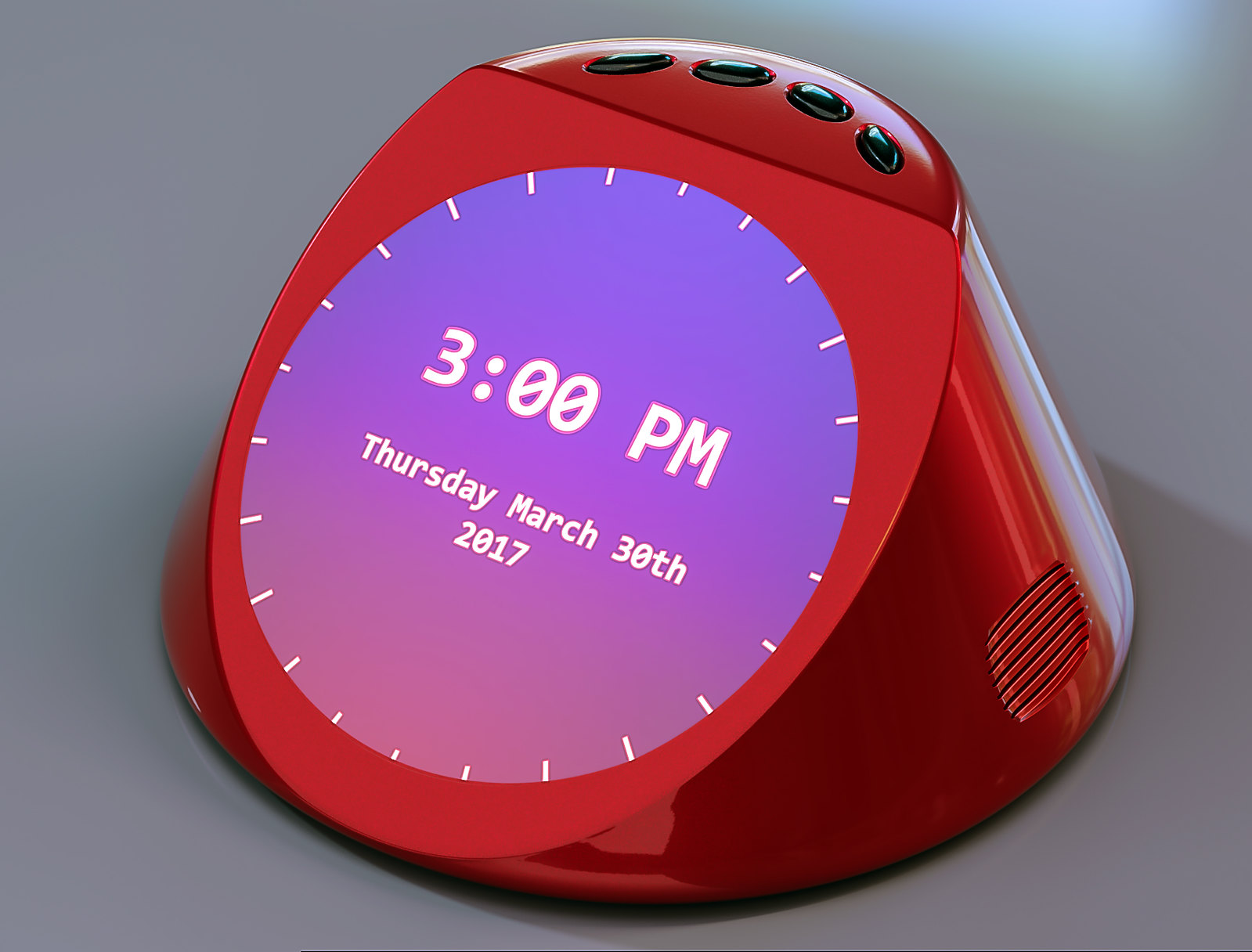The image depicts a large, photorealistic, computer-rendered clock set in a unique red housing. The housing is shiny, fire-engine red, and resembles a cone with its top sliced off at a diagonal angle, much like a carrot garnished. The overall shape is somewhat oval, akin to a toilet seat when viewed head-on, with the flat part at the top and rounded edges at the bottom.

The clock face is centrally located and digital, featuring a striking purple background with white digital text displaying "3 p.m." along with "Thursday, March 30th, 2017" directly below it. The digital display also has subtle white ridges extending downward in a circular pattern, enhancing its visual appeal.

At the top of the clock are four black buttons likely used for setting the time and alarm functions. On the bottom right side, there is a small red vent, possibly functioning as a speaker for the alarm sound to prevent overheating. The entire scene is set against a grey background that shows a gradient from dark grey at the bottom to a lighter shade towards the top left and right, accompanied by a shadow line that adds depth to the composition.